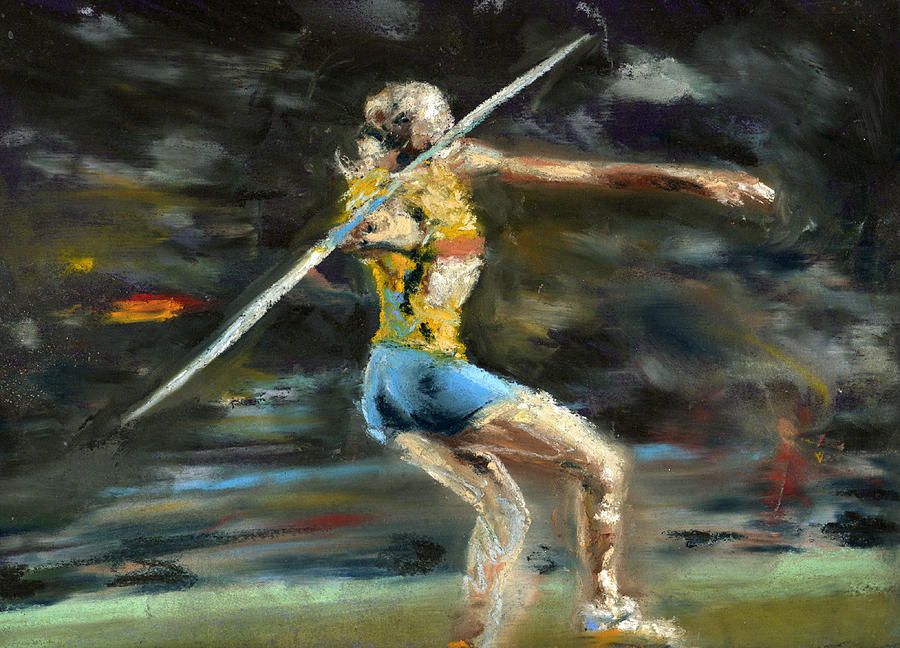This hand-painted color image is an impressionistic depiction of a female athlete in mid-motion, captured in an oil pastel or Monet-like brush stroke style. The artwork vividly portrays the athlete poised to throw a javelin, with her left arm extended horizontally in front of her and her right arm drawn back, gripping the javelin which has white tips and a blue shaft. She is dressed in a blue jersey and blue shorts, with some descriptions also noting a yellow jersey and red accents. Her blonde hair suggests it's a woman. The painting's background features a mosaic of blurred black, white, red, and blue smudges, emphasizing her dynamic motion. The soft transitions and abundance of varied brush strokes give the painting a fluid and somewhat distorted appearance, colorfully merging to vividly represent the scene.